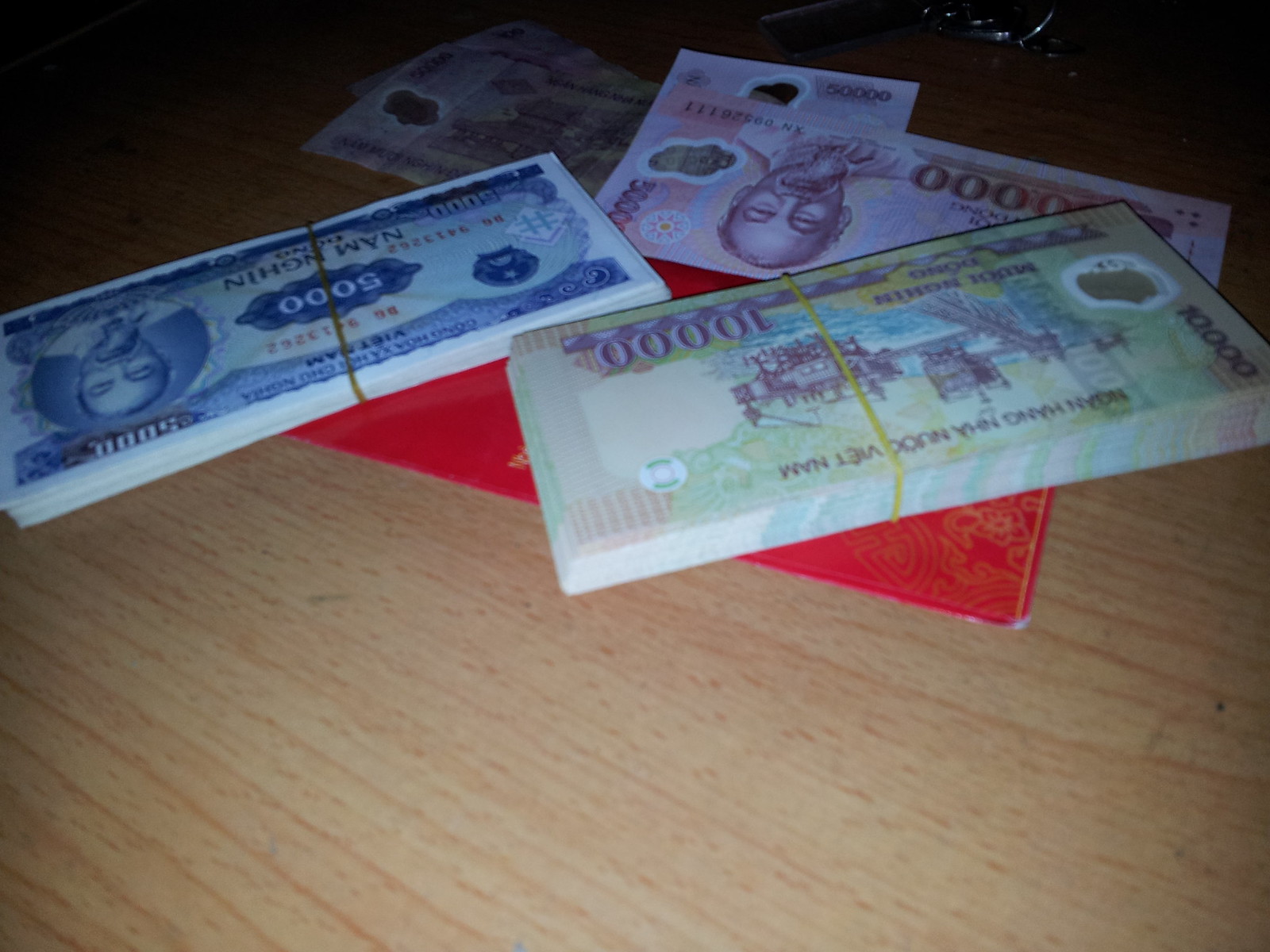The image depicts a collection of foreign currency laying on a light, creamy beige-brown wooden table. At the center of the photo are two prominently visible bundles of money, each secured with an elastic band. The first bundle, positioned at the left, features green bills marked with "10,000" and appears to showcase some scenery or buildings. Beside it, the second bundle consists of blue bills with the denomination "5,000" and includes a portrait of a man on the right side of the bills. Additionally, a partly visible purplish bill, located beneath the two bundles and slightly sticking out, also seems to depict the same man as on the blue bills, although the exact denomination is unclear. The image background is somewhat dim, making certain details less discernible, but there appears to be another bill with an indistinct denomination and another possible bill in shadow. At the very bottom, a red envelope or paper is tucked under these currency bundles, adding a splash of color to the composition.